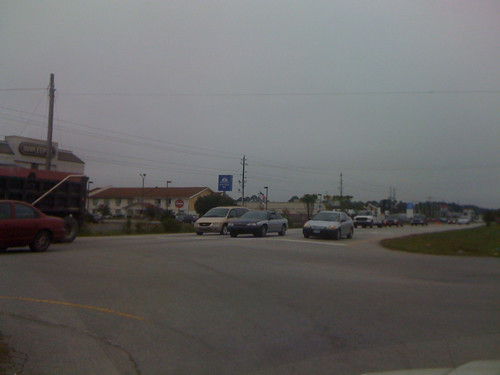In the image, taken in very low light during either a very dull day, early morning, or late evening, several cars are approaching a junction. The backdrop features a complex of buildings, including a long, possibly double-storey structure. To its left, there appears to be an industrial unit with a tall pole extending skyward. Multiple vehicles navigate the intersection, with one car specifically coming in from the left. The road meanders off into a densely built-up area in the background. The overcast sky casts a dreary, grey hue over the scene, which is mirrored by the road's even more muted grey. The only splash of color is a small patch of grass on the right, adding minimal contrast to the otherwise monochromatic landscape.